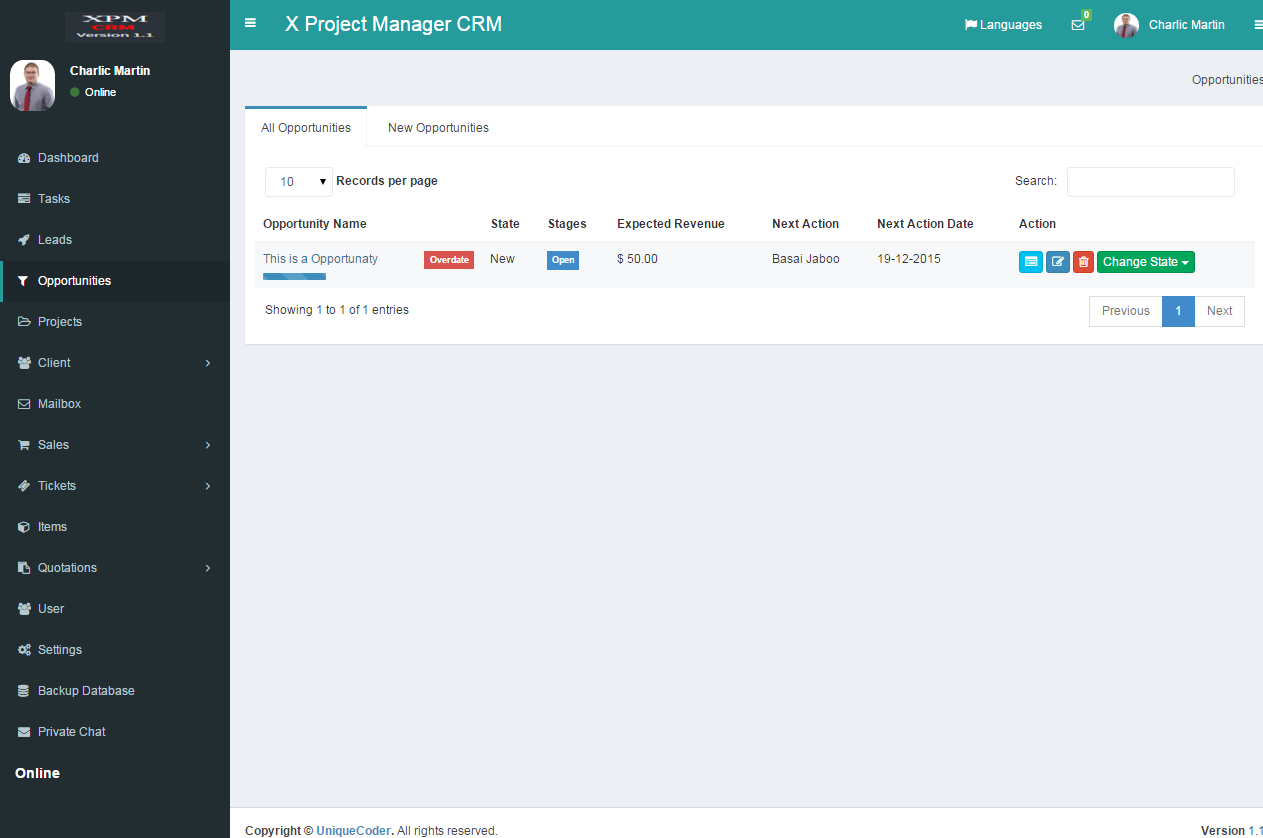This is a screenshot of a website interface for a CRM platform named "XPM CRM." On the left side of the screen, there is a vertical black sidebar. At the top of this sidebar, "XPM CRM" is displayed in white font, followed by the user’s name, "Charlie Martin," and a green circle indicating online status. To the left of the name and status, there is a small profile picture of Charlie Martin, who appears to be a middle-aged white man wearing a gray button-up shirt and a black tie, with a white background.

Below the profile section, there is a vertical menu listing various navigational options: Dashboard, Tasks, Leads, Opportunities (highlighted as the current selection), Projects, Clients, Mailbox, Sales, Tickets, Items, Quotations, User Settings, Backup Database, and Private Chat. At the bottom of the sidebar, the word "Online" is also displayed in white.

To the right side of the screen, the main content area is focused on "Opportunities," specifically showing a section titled "All Opportunities." Within this section, there is a white bar with a dropdown menu allowing the user to select the number of records displayed per page, currently set to "10 records per page." However, only one record is shown, labeled as "This is an opportunity."